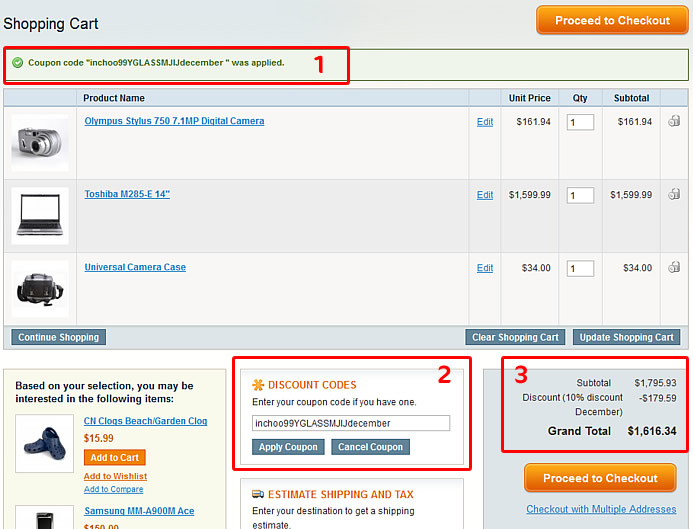The image depicted is a screenshot of an Amazon online checkout page with a bluish-gray background. In the top left-hand corner, the words "Shopping Cart" are prominently displayed. In the top right-hand corner, there's an orange button labeled "Proceed to Checkout" in white text.

Beneath these elements, there is a red box marked with a "1," indicating that a coupon code "INCHOO99YGLASSMJLJ December" has been applied.

Below this, the screen displays a grid with columns for product name, unit price, quantity, and subtotal. The grid lists three items:
1. **Olympus Stylus 750 7.1 MP Digital Camera**  
   - Unit Price: $161.94  
   - Quantity: 1  
   - Subtotal: $161.94

2. **Toshiba M285E14**  
   - Unit Price: $1,599.99  
   - Quantity: 1  
   - Subtotal: $1,599.99  

3. **Universal Camera Case**  
   - Unit Price: $34.00  
   - Quantity: 1  
   - Subtotal: $34.00  

At the bottom left of the screen, a blue button labeled "Continue Shopping" is visible. On the right-hand side, there are two buttons labeled "Clear Shopping Cart" and "Update Shopping Cart." 

Further down on the right-hand side, the discount codes are displayed, followed by the subtotal and grand total, which amounts to $1,616.34.